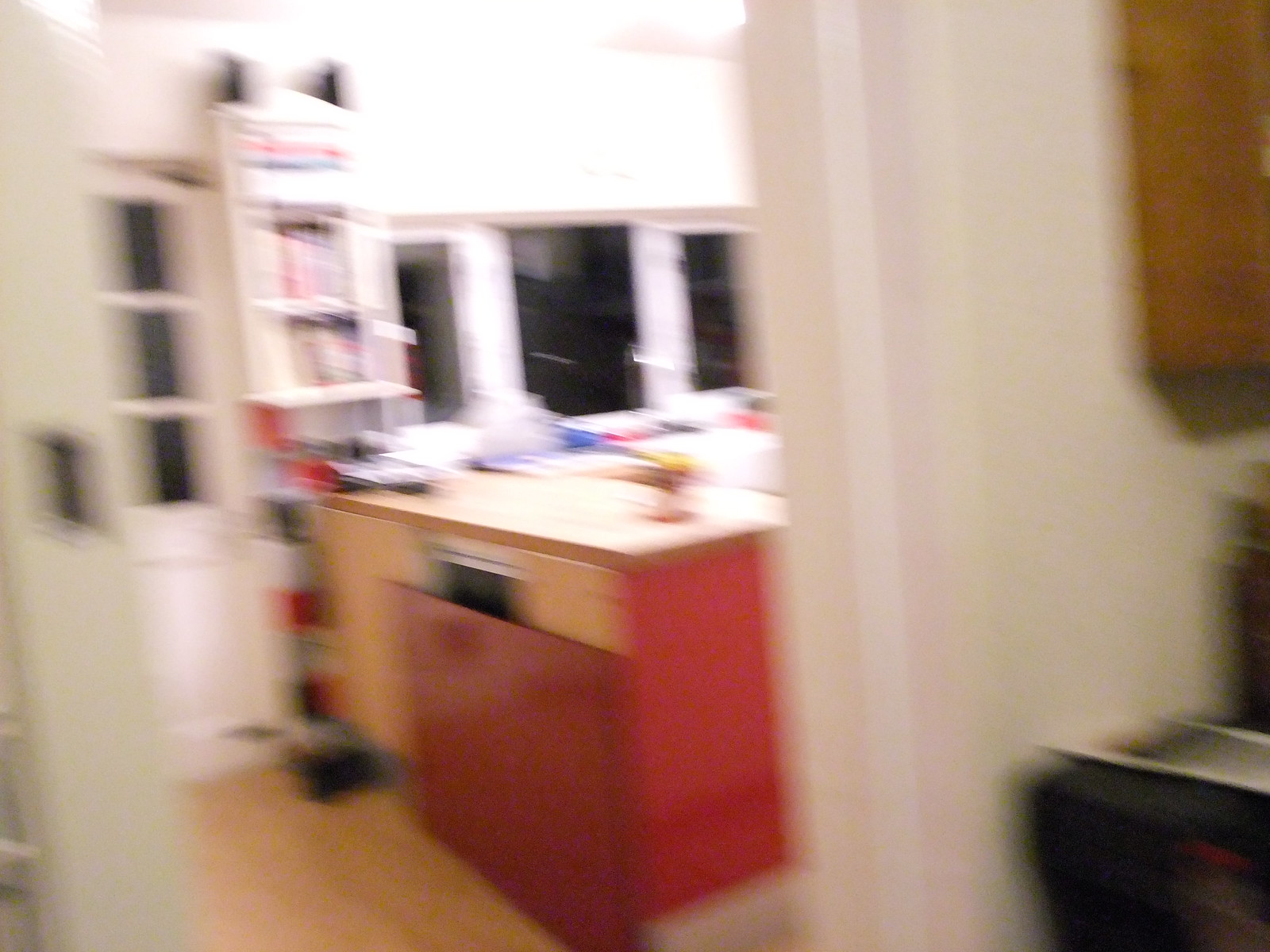This indoor photo is notably blurry. In the upper left corner, there's a door with windows positioned at the top. To the right of the door, a tall, floor-to-ceiling object is visible. Further right, there are three windows in a row. Positioned in front of these windows is a red cabinet with a white top. The flooring appears to be hardwood. Adjacent to this, there is another doorway bordered by a wall on its right side. There is also an unidentified object resting to the right of this doorway, accompanied by another wooden item mounted on the wall nearby.